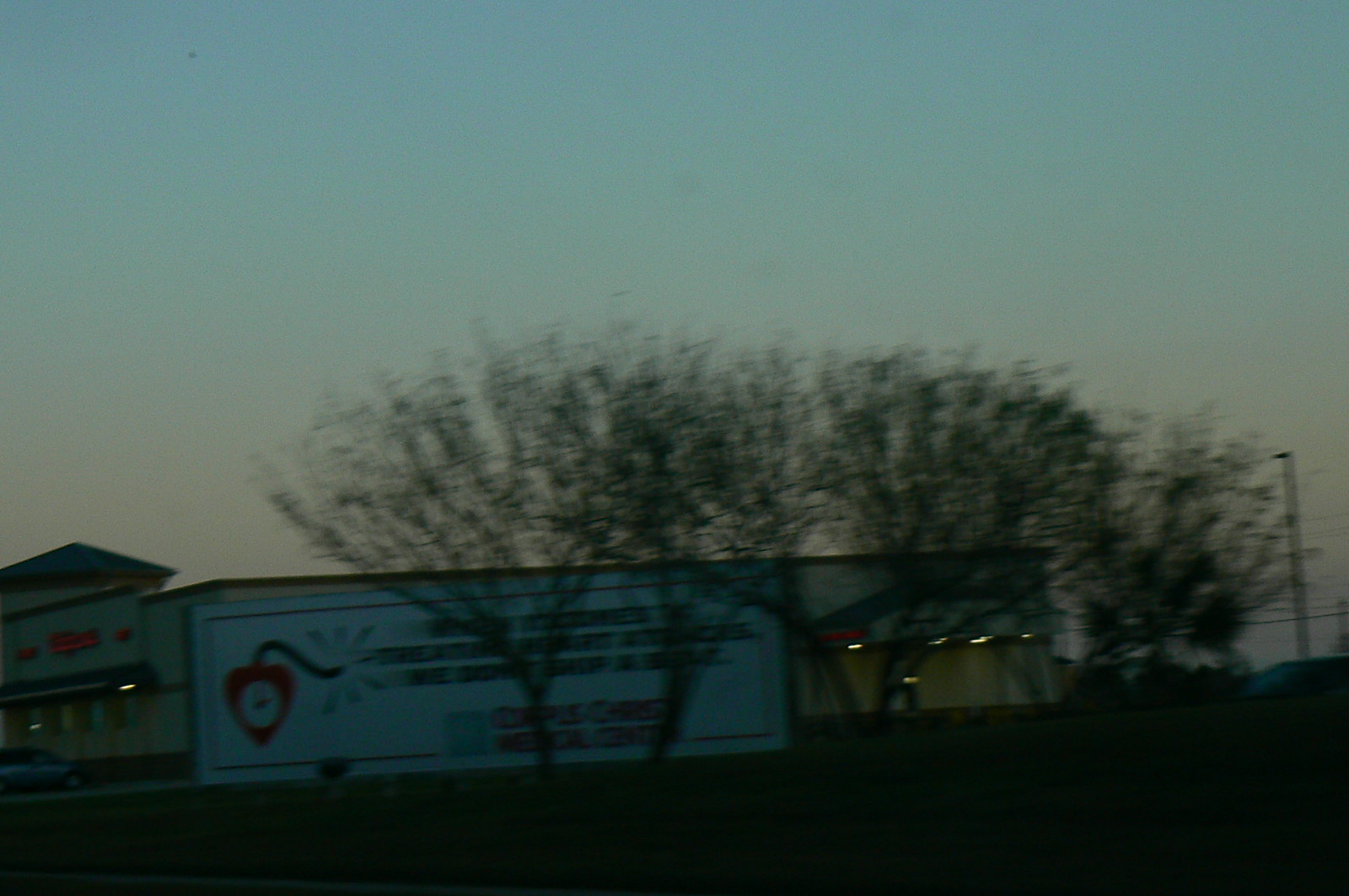A blurry, dusk-lit photo captures the exterior of a Walgreens, partially obscured by shadowy, leafless trees. The image, taken from a grassy field adjacent to the store, reveals an indistinct white sign beyond the trees, possibly indicating a nearby medical center with a faint heart symbol. The overall scene is cloaked in the twilight's dimness, adding to the photo's hazy and unfocused appearance.